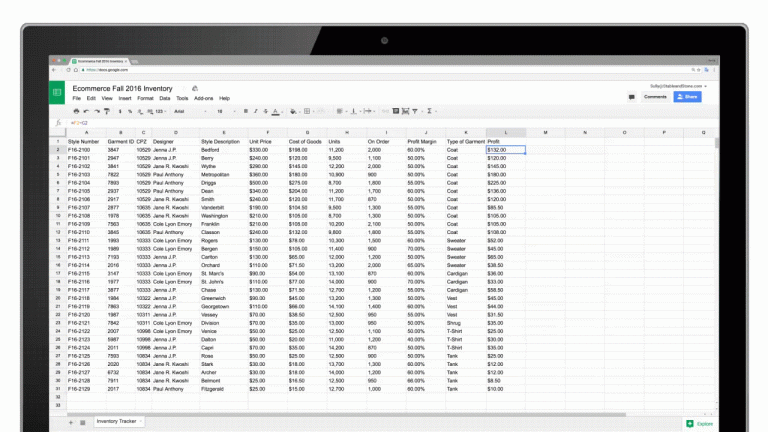The image is a horizontally aligned rectangular screenshot of an open Excel spreadsheet bordered in solid black with a hint of gray blended at the top. It showcases a table titled "e-commerce fall 2016 inventory," with columns spanning from A to L and filled with data across 21 rows. The spreadsheet headings include "store number," "garment ID," "designer," "style description," "department," "unit price," and various other categorical descriptors, though some are hard to decipher due to the image's blurriness. Despite the difficulty in reading the finer details, it is evident that the spreadsheet contains detailed information pertaining to an e-commerce inventory for fall 2016. The cells are populated with numbers, letters, and words, indicating inventory details such as designer names, quantities, and prices. In the bottom corners, additional labels are visible, with "inventory tracker" on the left and "explore" on the right. The image is colorful and clear, aided by natural lighting, although the precise details remain challenging to read.